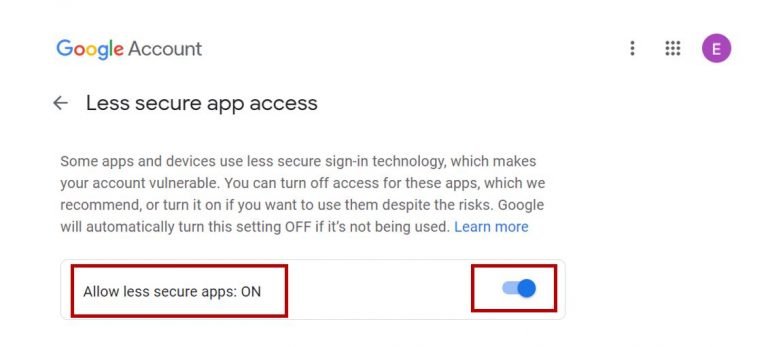**Descriptive Caption:**

The image is a screenshot from a Google account settings page. At the top, the recognizable "Google" logo is displayed in its iconic multicolored letters. To the right of the logo, "Account" is written in plain black text. Below this header, there is a left-pointing arrow next to the phrase "Less secure app access" indicating navigation or a previous section.

Moving further down, a blank area precedes an informative text section. The text explains that some apps and devices use less secure sign-in technology, making the account vulnerable. It suggests turning off access for these apps to protect the account, although users can choose to turn it on despite the associated risks. Google indicates that it will automatically turn this setting off (emphasized in all capital letters: "OFF") if it remains unused. This entire message is in black print.

Alongside this text, there is a blue hyperlink labeled "Learn more" for additional information. As the viewer's eyes travel further down, a faint gray rectangle becomes visible, enclosing the bottom portion of the screenshot.

Inside this gray rectangle, there are two red rectangles. The first red rectangle contains the text "Allow less secure apps: On" next to a blue toggle switch that indicates the setting is activated and currently turned on.